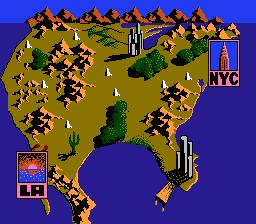This image is a screen capture from a computer game, showcasing an aerial view of a simplified, topographical map of North America. The map spans from Upper Canada down to the fringes of Central America. Prominent features include tall mountains dominating the upper region in Canada, with smaller mountain ranges scattered throughout the landscape. Verdant green areas punctuate the map, indicating forests or plains. In the Florida Panhandle, a striking cluster of skyscrapers suggests significant urban development. A solitary cactus marks the approximate location of Arizona, adding a touch of the desert environment. The lower left corner of the map is labeled "LA," representing Los Angeles, while the upper right corner bears the label "NYC," designating New York City.